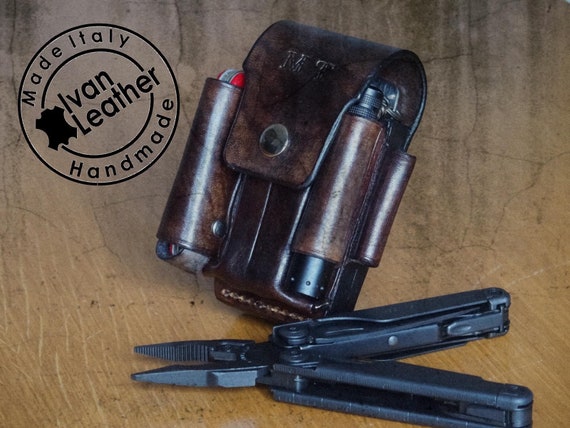This detailed advertisement showcases a meticulously crafted, dark brown leather pouch by Ivan Leather, prominently displaying the initials "MT" on its flap and secured with a button. The pouch, handmade in Italy as indicated by the circular "Made in Italy, Handmade" badge in the top left corner, is designed to hold multiple tools and accessories. Inside the pouch, a black Leatherman multi-tool with pliers stands out against the traditionally silver models, accompanied by a Swiss Army knife and a small flashlight. The items rest on a brown wooden table with a distinctive crackled finish, emphasizing the artisanal quality of both the tools and the leather pouch.